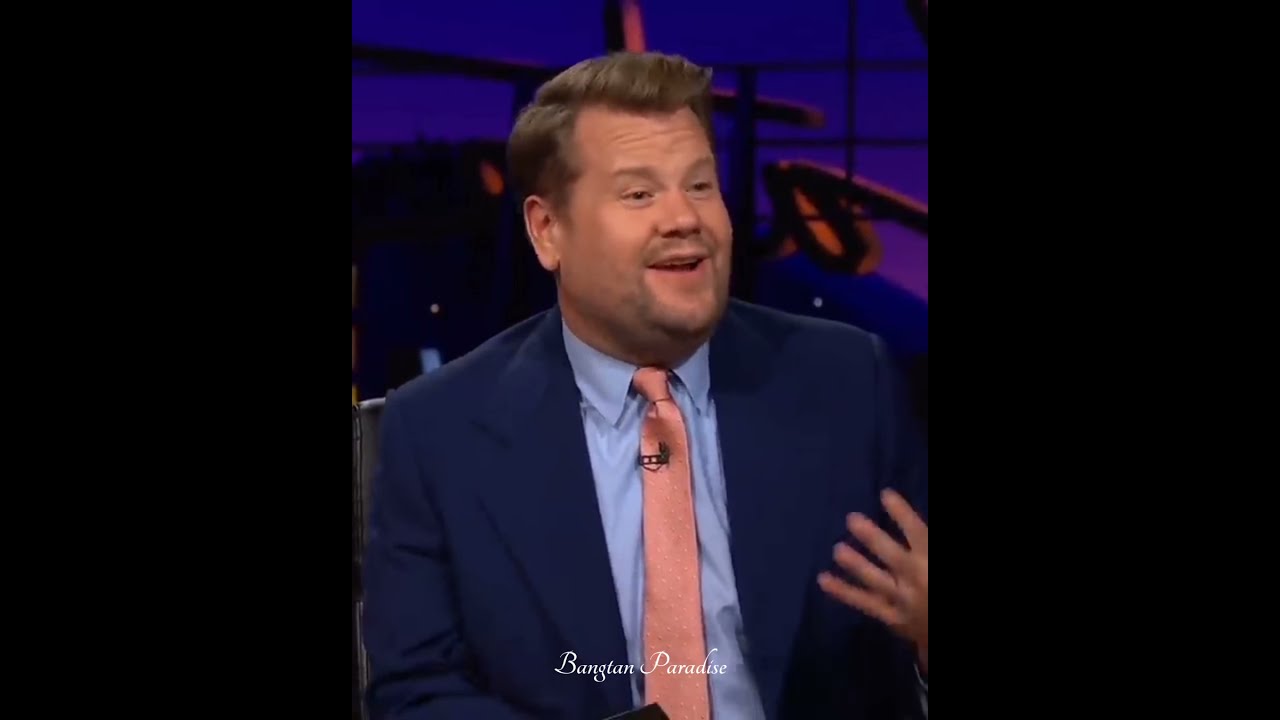This full-color photograph, taken by Bunglan Paradise, captures late-night talk show host James Corden in the midst of an animated moment on set. The horizontally rectangular image is dominated by a thick black border on both sides, framing Corden centrally. He is well-dressed in a darker navy blue jacket paired with a light blue button-up shirt, accessorized by a salmon, or pinkish coral tie, to which a microphone is clipped. Corden, a man in his 30s with sandy blonde, wavy hair, and a few days' growth of a goatee, is captured mid-speech, his mouth open slightly, revealing his top row of teeth, and his left hand gesturing expressively. The backdrop appears to be indistinct but hints at a blue-lit setup typical of his late-night show environment. This expressive photograph highlights Corden's signature flair as he engages in what appears to be a lively commentary.